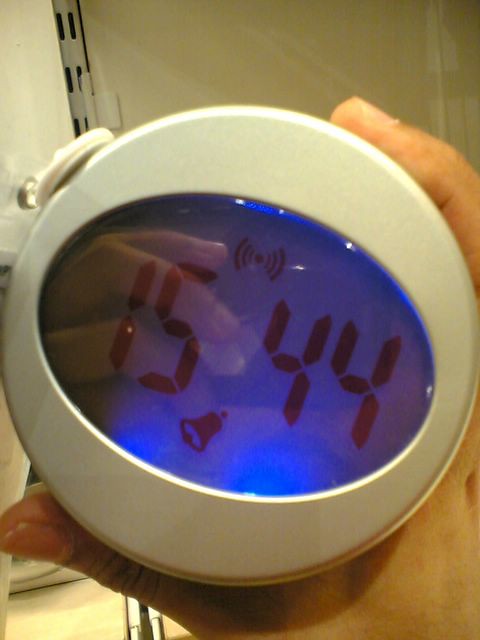This image showcases a hand-held alarm clock, slightly tilted to the right, displaying the time 15:44. The clock features a blue oval face set within a thick, round white casing. A person's pinky finger or thumb is visible at the top right edge of the clock, suggesting they are holding it. The background reveals a white wall and, to the left, gray shelving slots. A piece of paper appears to be taped over the shelving, with a visible strip of tape running down the side and onto the wall, partially peeling off.